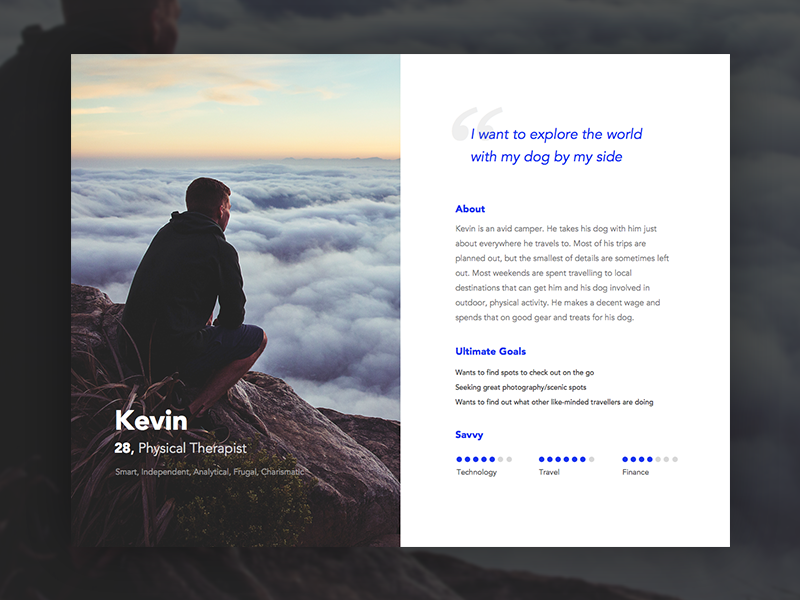In this image, we see a photograph on the left side featuring a young white male named Kevin, who appears to be 28 years old. Kevin is seated on a rock, gazing thoughtfully into the distance. He has blonde hair and is dressed in a black sweater, black shorts, and black shoes. The text beneath his picture identifies him as a physical therapist, and describes his personality with words like "smart," "independent," "analytical," "frugal," and "charismatic."

To the right of the image, at the top middle, there is a statement written in blue text that reads: "I want to explore the world with my dog by my side." Below this statement is a section titled "About," providing more details about Kevin. It explains that Kevin is an avid camper who enjoys taking his dog along on his travels. While most of his trips are meticulously planned, he often leaves room for spontaneous adventures.

Further down, there is another section labeled "Ultimate Goals." This part outlines Kevin's aspirations, stating that he wants to discover new places on the go, seek out scenic spots for photography, and learn what other like-minded travelers are doing. At the very bottom, additional interests are listed: "savvy in technology, travel, and finance."